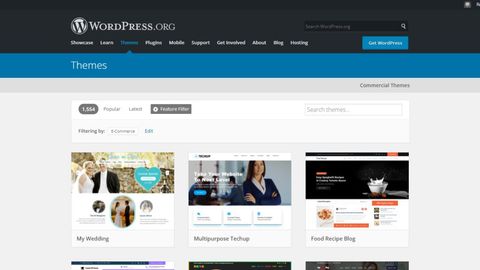The image displays a slightly blurry webpage identified as WordPress.org at the top. The layout is characterized by a black navigation bar with various sections, including "Showcase," "Learn," "Themes," "Mobile," "Support," "Get Involved," "About," and another unreadable section. There is also a prominent blue button labeled "Get WordPress," suggesting the website's purpose of encouraging users to utilize WordPress services.

Below the navigation bar, several WordPress theme examples are showcased. These include a wedding theme, a multi-purpose tech startup site, and a food recipe blog, each illustrating the diverse applications of WordPress themes. The overall design features a predominantly gray background, complemented by blue and black bars, providing a structured and visually appealing layout.